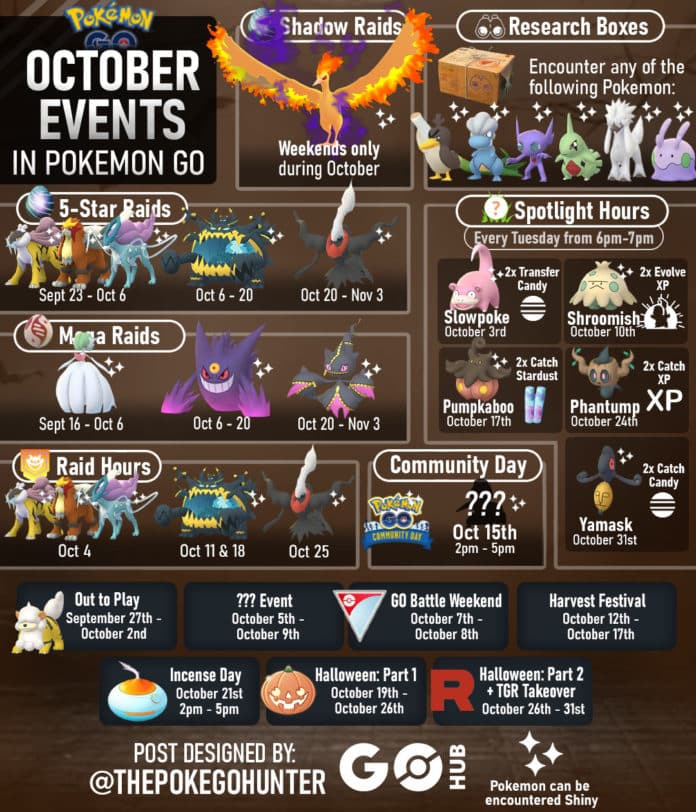Detailed Banner Caption:

"This vibrant banner advertises the October events in Pokemon Go. In the top left, the iconic Pokemon Go logo is prominently displayed, partially overlapping with bold text that reads 'October Events in Pokemon Go.' To the right of this, in a pill-shaped outline, is 'Shadow Raids,' featuring an image of the majestic Phoenix Pokemon. It highlights that these raids are available 'Weekends only during October.' Further right, another pill-shaped outline spotlights 'Research Boxes,' inviting players to 'Encounter any of the following Pokemon,' with six different Pokemon images displayed below. Directly beneath this main section is another pill-shaped outline marked 'Five Star Raids,' showcasing a trio of Pokemon with specific dates listed underneath, followed by two individual Pokemon, each with their respective dates."